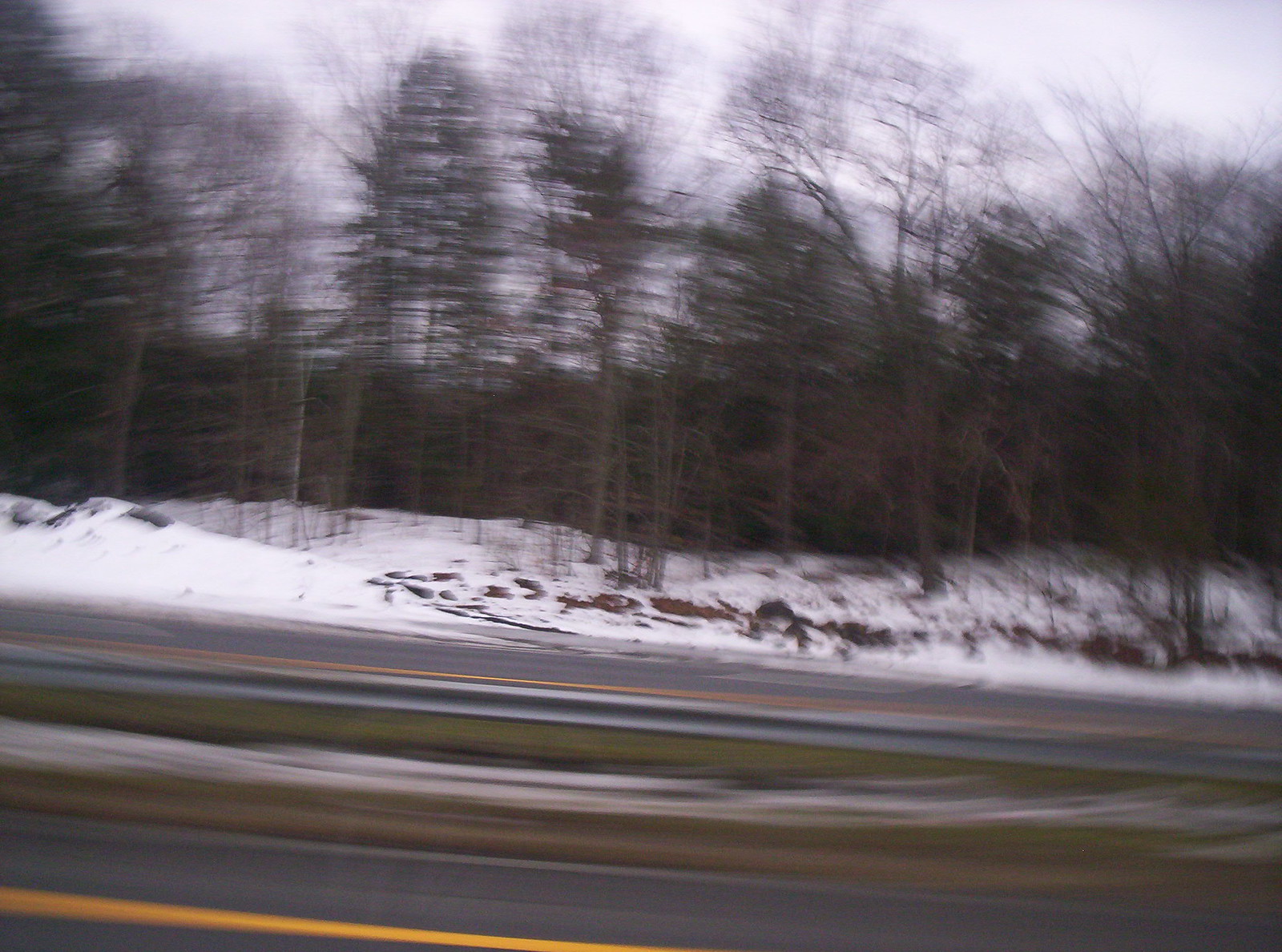The photograph is a horizontally-oriented, slightly rectangular image, captured from a moving vehicle, resulting in a noticeable blur. The frame spans multiple empty lanes of traffic, with no vehicles present. The scene includes a center grassy median that dips slightly towards the bottom right of the image. Dominating the upper portion of the frame is a hilly expanse shrouded in snow, on the far side of the road. This area is densely populated with numerous straight trees, some of which retain a few leaves, though most stand barren. The overall blur impacts the clarity of the trees and the snowy hillside, contributing to a sense of motion and fleeting observation.